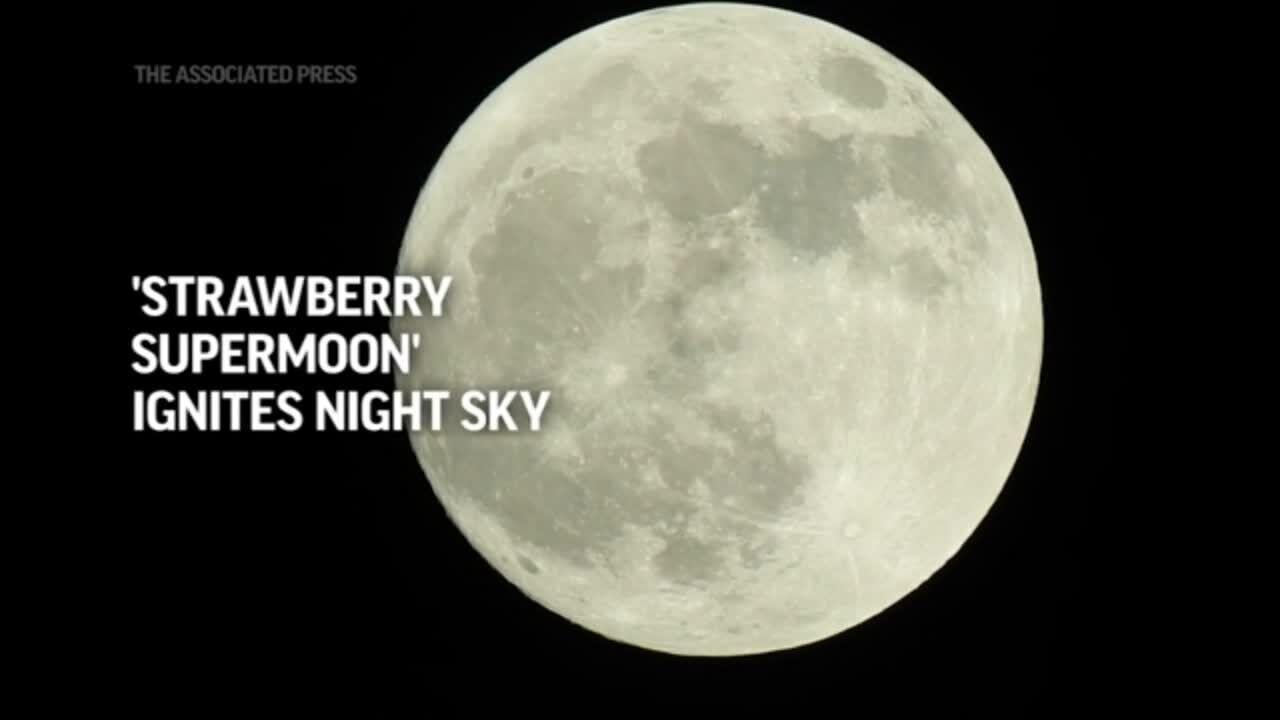This rectangular poster features a solid black background dominated by a bright, full moon in the center, showcasing its surface features with darker gray splotches and lines of white and pale gray. In the upper left corner, there is faint white text reading "The Associated Press," almost like a watermark. To the left of the moon, written in large, bold, white letters, it says, “Strawberry Supermoon Ignites Night Sky," with "Strawberry Supermoon" in quotation marks. The ends of the words "Sky" and "Strawberry" overlap slightly with the moon's image, adding to the depth and intrigue of the poster.